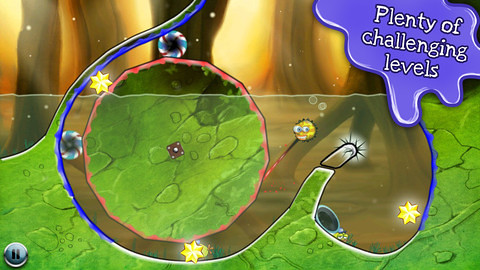The image depicts a vibrant and engaging video game interface with a landscape that is wider than it is tall. In the upper right-hand corner, white text against a purplish-blue, ink-like backdrop proclaims "Plenty of challenging levels." Below a defined waterline sits a prominent green structure, set against an abstract background characterized by vertical bands of brown and yellow hues. Scattered throughout the water and above are various icons including a sinister, little demonic face, glowing yellow stars, and candy cane-striped life preservers. A possible die rests in the middle of a circular green shape, while a small pause button can be found in the lower left-hand corner of the screen. This colorful and dynamic scene suggests a computer game designed for younger players, offering visually appealing elements and interactive challenges.